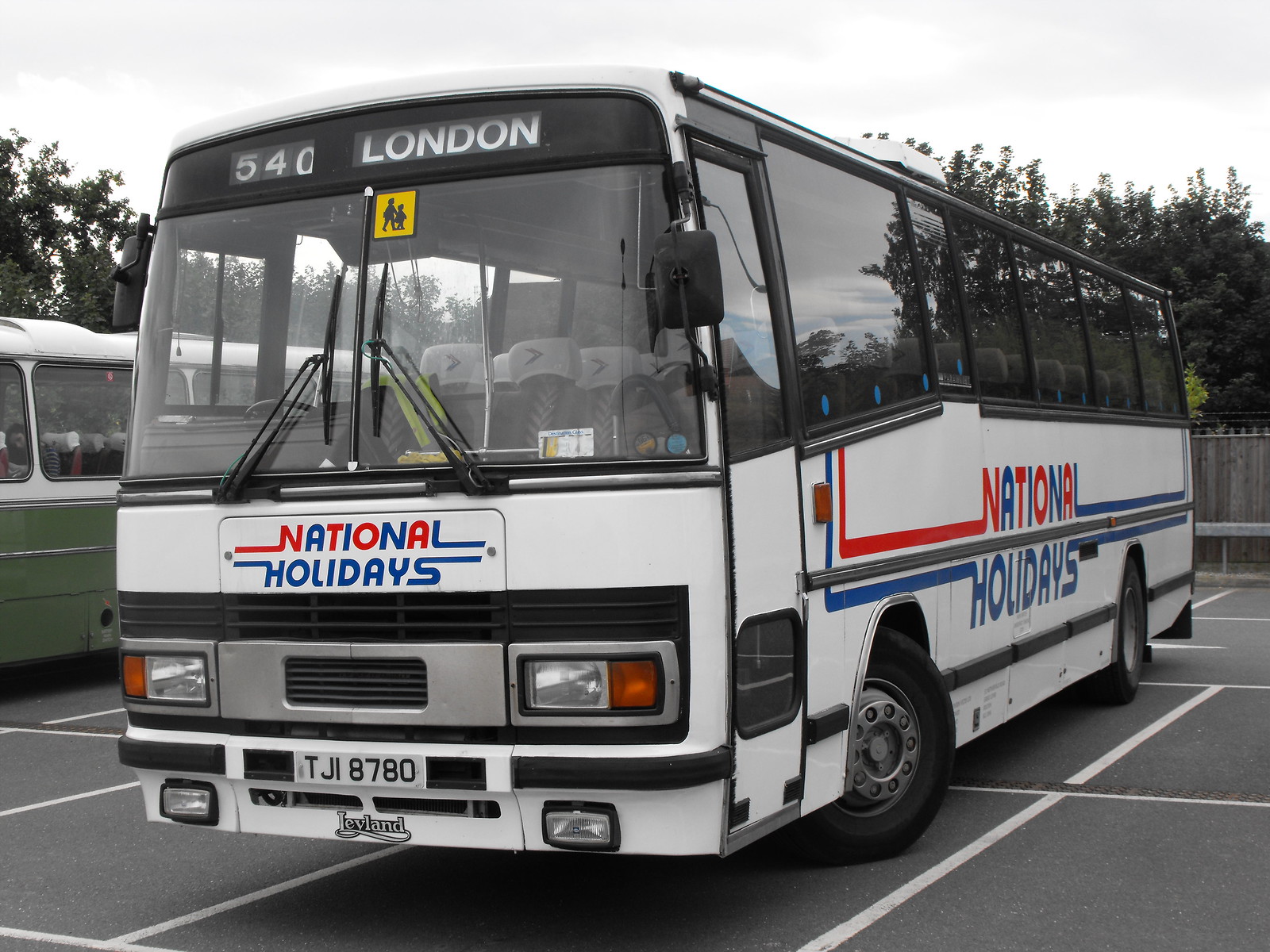The image depicts a white bus parked in a spacious, dark gray, paved parking lot with thick white painted borders. The bus, identified as a Leyland model, has its front facing left and extends into the distance towards the right. The front top of the bus prominently displays "540 London" in white letters, while below the driver's window and on the side of the bus, the text "National Holidays" is written in alternating red and blue letters. The license plate reads TJI 8780, and beneath it, there's a Loveland logo. The bus features gray fabric patterned seats visible through its windows. Behind this vehicle, to the left, is another bus colored green and white, where a girl with black hair, dressed in a black and white striped shirt, is seated against a red chair. The backdrop reveals overcast skies and the tops of some trees.